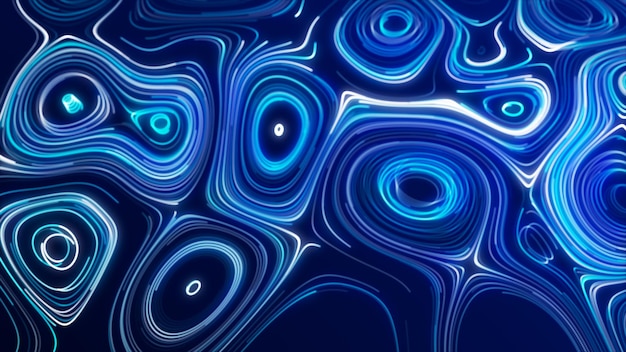The image depicts an elaborate and abstract digital design set against a very dark blue, almost navy background. The artwork features an intricate pattern of spiraling, swirling shapes resembling distorted circles and fractals, reminiscent of microscopic views of sliced bacteria or the natural rings found in geodes and agates. The varying shades of blue—ranging from very light sky blue to medium electric hues and occasional white highlights—create a glowing, neon-like effect that gives the design a luminescent quality. Some of the spirals intersect, though none overlap completely, and a few even contain bright red circles at their centers, adding a striking contrast. This intricate, computer-generated tapestry of interconnected shapes and colors offers a mesmerizing visual experience, with its layers of light and dark blues swirling together to form an aesthetically pleasing abstract composition.